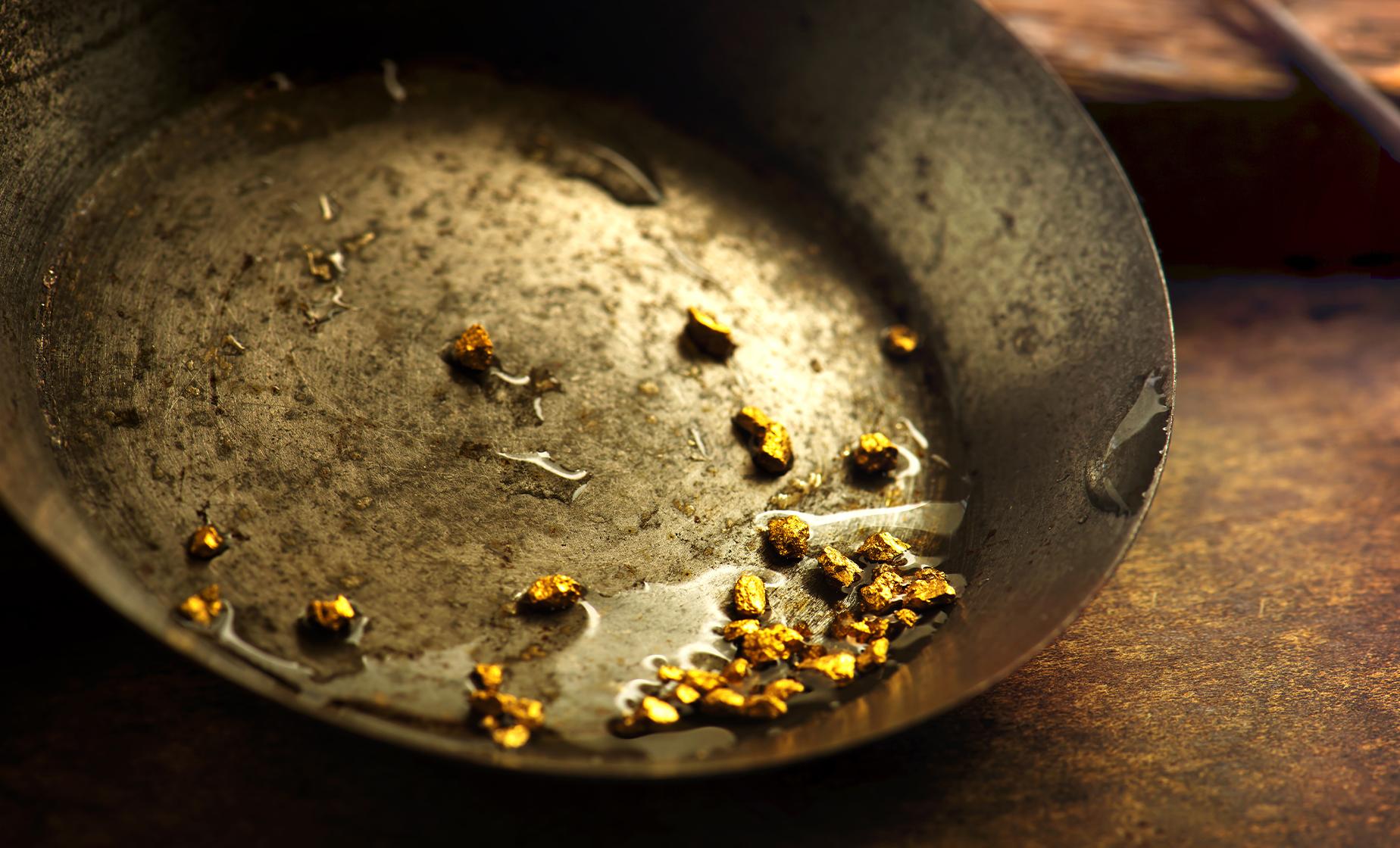In this landscape-oriented close-up photograph, a well-worn, metallic-grey pan is prominently displayed, positioned towards the center-left of the image and tilted slightly. The pan contains clear water, in which numerous tiny, glistening gold pellets are clustered. The gold, strikingly yellow, contrasts sharply against the dull metallic sheen of the pan and the clarity of the water. The surface beneath the pan appears rough and brown, possibly rusted, complementing the pan's aged and grimy appearance. To the upper right corner, a blurred stick-like object can be seen. The background and corners of the image are dark and blurry, with hints of brown, further focusing attention on the luminous gold within the pan’s clear liquid.